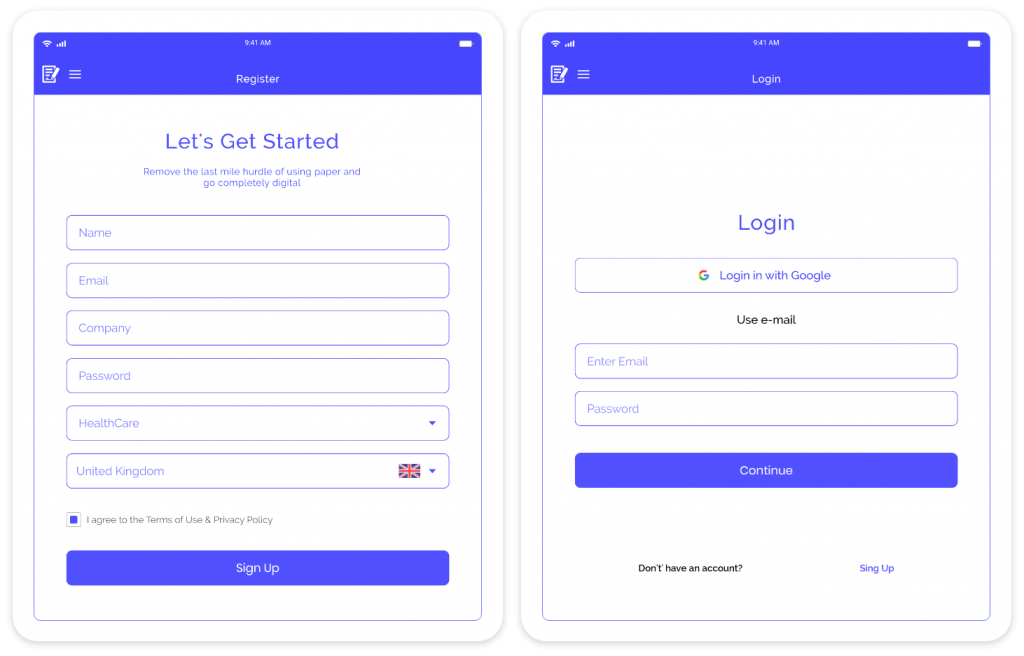The screenshot features a registration screen for an application with a bright violet background that is difficult on the eyes. The foreground includes voice text instructions overlaid on a white background. At the top, there's a field labeled "Name," though the text beneath it is unreadable. The overall interface design mirrors the violet text against the white background.

Prominently, the form fields include "Name," "Email," "Company," "Password," and the user's jurisdiction or industry-related input such as "Healthcare" and "United Kingdom." Below these fields, users are prompted to agree to the "Terms of Use" and "Privacy Policy," accompanied by prominently colored buttons for signing up.

To the right of the sign-up section, there are options to "Login" or "Login with Google," followed by fields for entering email and password. A large "Continue" button is situated beneath these login options. At the bottom of the screen, an invitation to create a new account reads, "Don't have an account?" with a "Sign Up" link in bluish text on a white background.